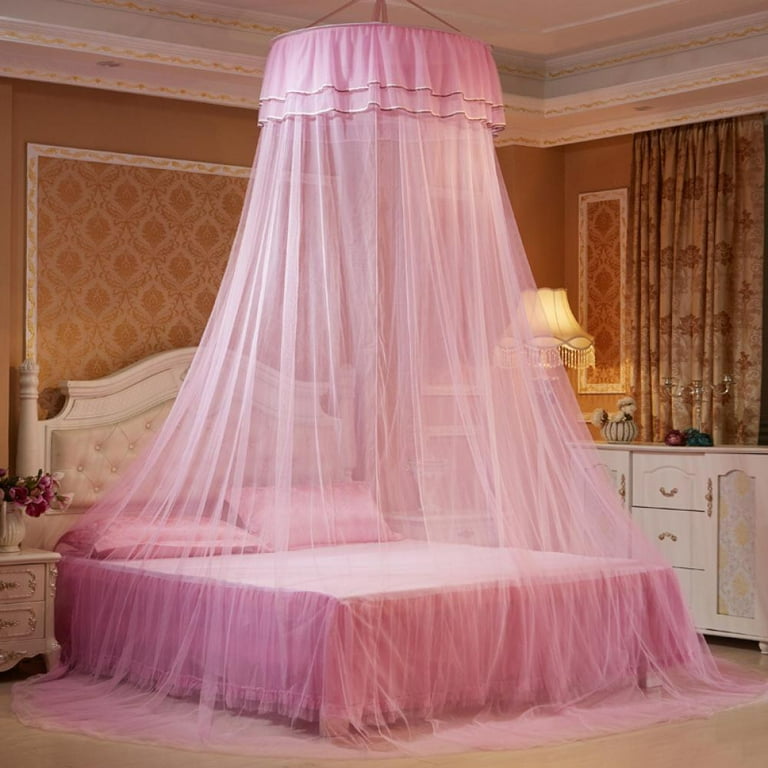The photograph depicts a cozy and well-decorated bedroom interior, featuring a harmonious blend of pink, white, and brown tones. At the center, a bed is adorned with pink sheets and pillows. Draping from the ceiling, a delicate pink mosquito net made of sheer tulle flows gracefully down to the floor, enveloping the bed in an ethereal canopy.

The headboard, placed against the left wall, is white with a raised, padded central area accentuated by pale yellow fabric and little beveled circles. Flanking the bed are nightstands; the one on the left holds a white vase with pink flowers, adding a touch of nature and color to the room.

To the right side of the image, there's a piece of furniture - either a shelf or chest - featuring white drawers that ensure additional storage. Potted plants or vases sit atop this cabinet, enhancing the room's fresh and natural ambiance.

The walls are adorned with brown wallpaper, incorporating a repeating pattern that enriches the room's elegance. Beige and brown curtains hang on the right, complementing the light brown flooring. The ceiling is recessed and bordered with a white trim, adding an element of architectural interest.

A switched-on shade light in the corner softly illuminates the room, casting a warm and inviting glow over the thoughtfully designed space.